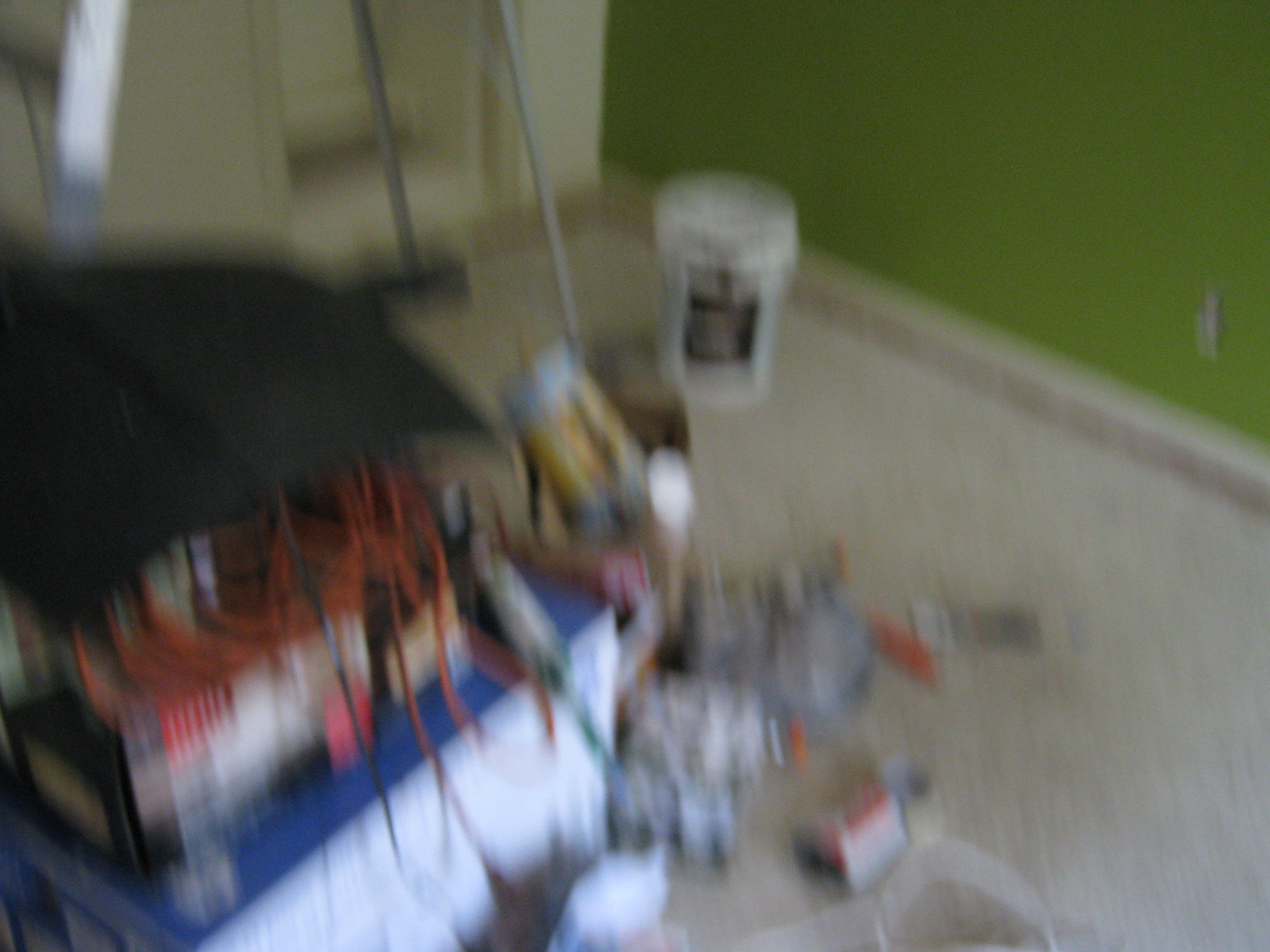This image features a cluttered and chaotic scene. On the right side, there's a wall painted an unattractive split pea green. In the upper left corner, a white tub is visible. The middle of the image is dominated by a floor covered in various indistinguishable items, adding to the messy appearance. Toward the lower left, there appears to be a stack of either boxes or electrical components, with noticeable orange wiring visible in the background. Additionally, a silver broom is propped against the wall in the upper portion of the image. The photograph is blurry, making it challenging to discern specific details.